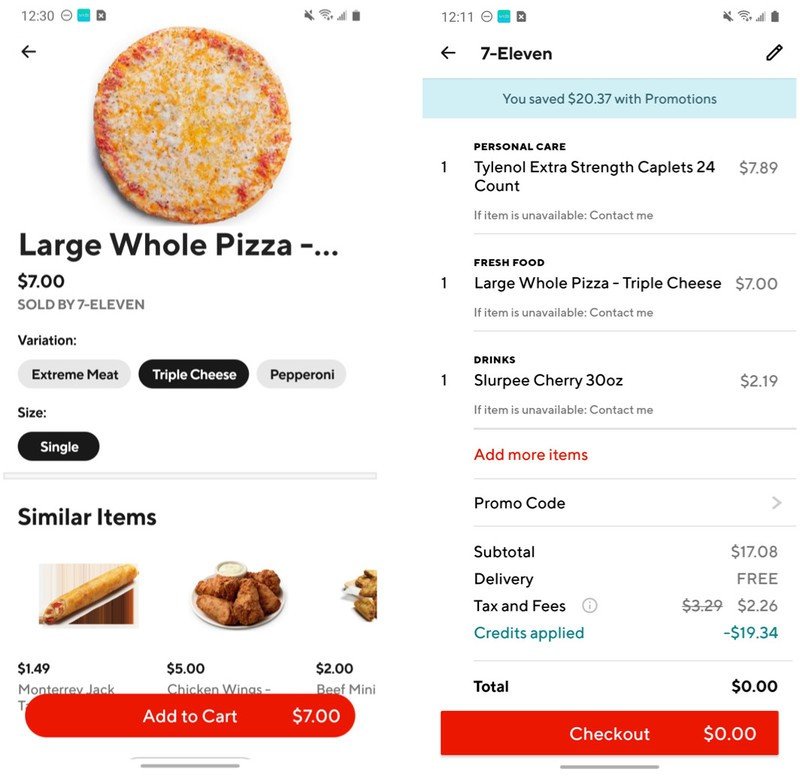The image showcases two screenshots from a smartphone displaying a 7-Eleven shopping app. 

The first screenshot is taken at 12:30 PM with a notable battery life remaining. It features a description for a large whole pizza priced at $7.00. The chosen variation is "Triple Cheese," with other selectable variations including "Extreme Meat," "Triple Cheese," and "Pepperoni." Below this section, there is a list of similar items, which includes Monterey Jack something, chicken wings for $5.00, and beef minis priced at $5.00 or $2.00. Each item is accompanied by an "Add to cart" option. 

The second screenshot continues with items available from 7-Eleven. It lists "Tylenol Extra Strength Caplets, 24 count" for $7.89, a large whole pizza for $7.00, and a "Slurpee Cherry, 30 ounces" for $2.19—all of which have been selected. An option to "Add more items" is visible in red, along with a promo code section that hasn't been utilized. 

The breakdown of costs shows a subtotal of $17.08, with free delivery, taxes and fees amounting to $2.26, and a credit of $19.34 applied. The final total is $0.00, indicating that the user has successfully obtained all items without incurring any costs, ready to proceed to checkout.